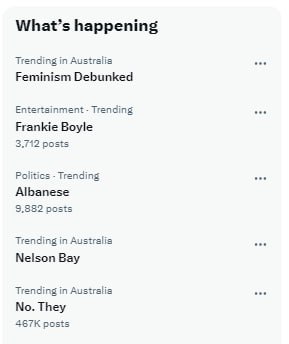This image appears to be a screenshot of a social media or news trend summary with a white background and bold black text, making it very clear and easy to read. At the top of the image, the heading "What's Happening" is prominently displayed. Beneath this, each trending topic is listed with a series of three black dots next to them, indicating bullet points.

- The first trend listed is "Trending in Australia: Feminism Debunked."
- Following that is "Entertainment Trending: Frankie Boyle" with 3,712 posts.
- Next is "Politics Trending: Albanese" with 9,882 posts.
- Another topic is "Trending in Australia: Nelson Bay."
- Finally, "Trending in Australia: No They" with a staggering 467,000 posts.

The text sits within a subtle gray box, enhancing its visibility. Although the black dots are slightly blurry and the font is mildly grainy, both elements remain highly legible, making the image accessible even for individuals with low vision. There are no additional images or decorative fonts; the focus remains entirely on the text, which is clean, straightforward, and bold.